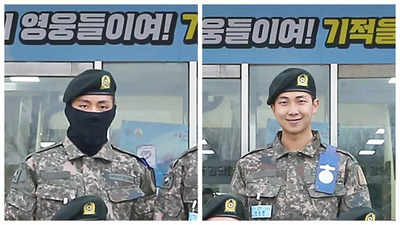The image depicts two Asian military men standing side by side in front of a building with large glass windows and foreign lettering in the background. Both are dressed in similar camouflage uniforms and wear berets, indicating they are part of the same or similar military unit. The soldier on the left has his face covered with a black cloth, leaving only his eyes visible, while the soldier on the right is smiling with no face covering. The latter also has a badge on his uniform, highlighting a difference between the two. The image is clear and well-lit, showcasing the detailed features and uniformity of the soldiers.